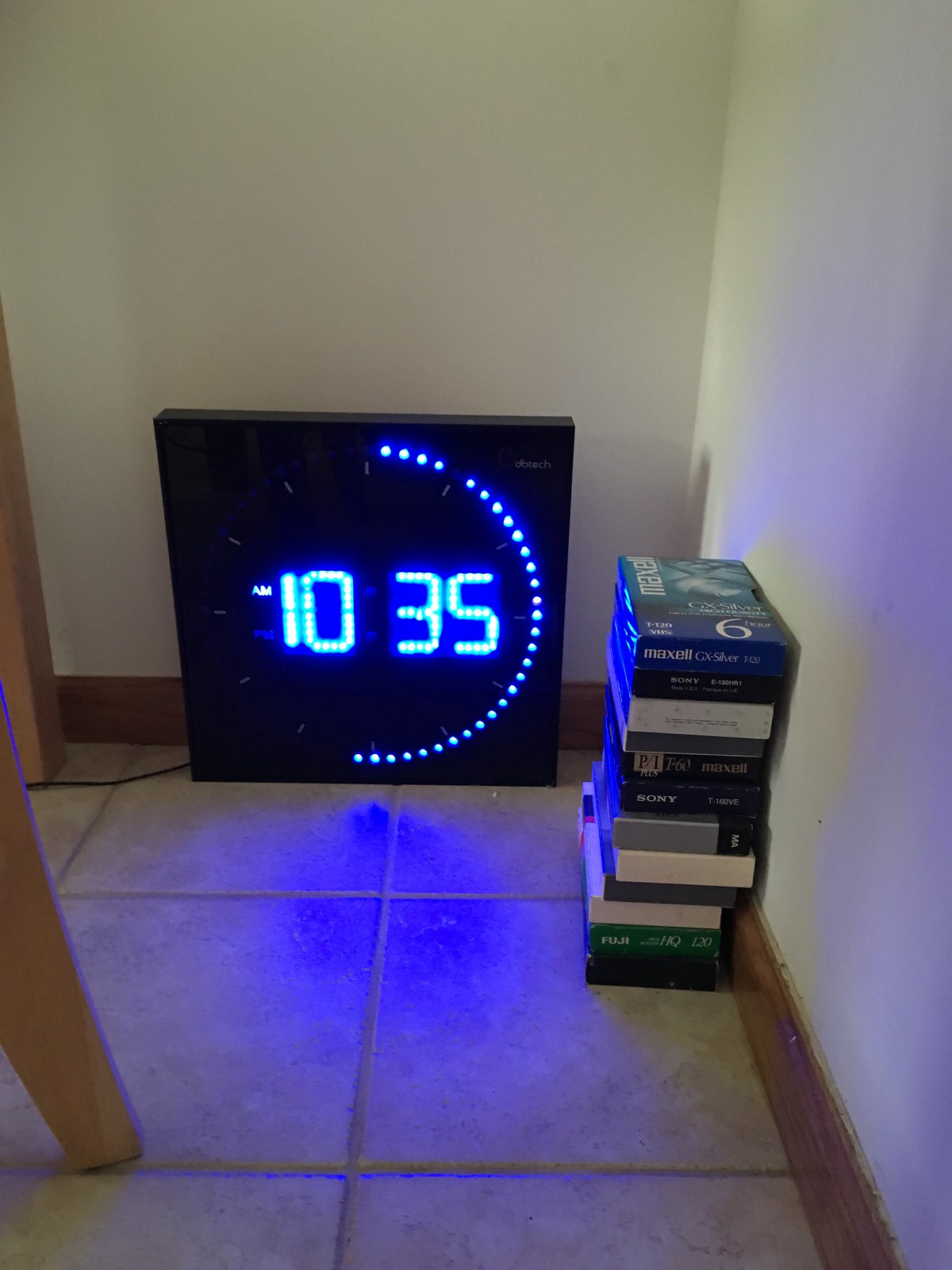A square, digital clock displaying "10:35 a.m." in bright blue fluorescent numbers is positioned on the floor in the corner of a room. The clock is oriented towards the camera, leaning against the back wall. To the right of the clock, old VHS tapes are neatly stacked, with their spines facing the left, aligned against the right wall. On the left-hand side of the image, a small portion of a chair's legs and what appears to be a leg of a table are visible, hinting at the presence of more furniture just outside the frame. The overall scene suggests a cozy, nostalgic corner, blending modern and vintage elements.